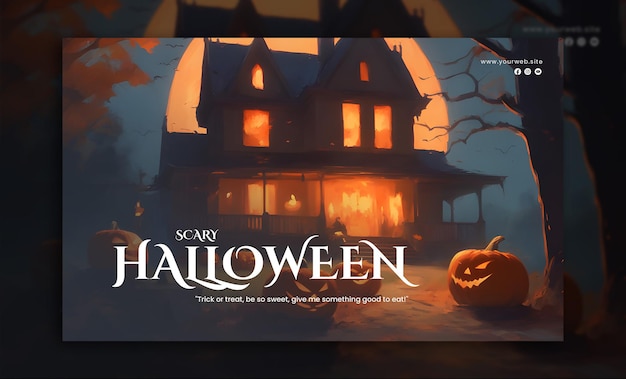The image is a screenshot from a web page, www.yourweb.site, featuring social media buttons for Facebook and Instagram along with another unidentified social button. The main graphic is a cartoon illustration set at night, showcasing a dark sky filled with flying birds or bats. The scene includes dark trees, some with leaves and others bare, adding to the eerie atmosphere. Central to the image is a spooky farmhouse, possibly two or three stories high, illuminated with an orange glow. Behind the farmhouse, there is a large, orange celestial body, either a sun or moon. The farmhouse, characterized by its wraparound porch, exudes an ominous and dark vibe. White text overlays the scene, reading: "It's a scary Halloween. Trick or treat, be so sweet, give me something good to eat." Completing the Halloween theme is a lit jack-o-lantern, enhancing the overall spooky ambience.